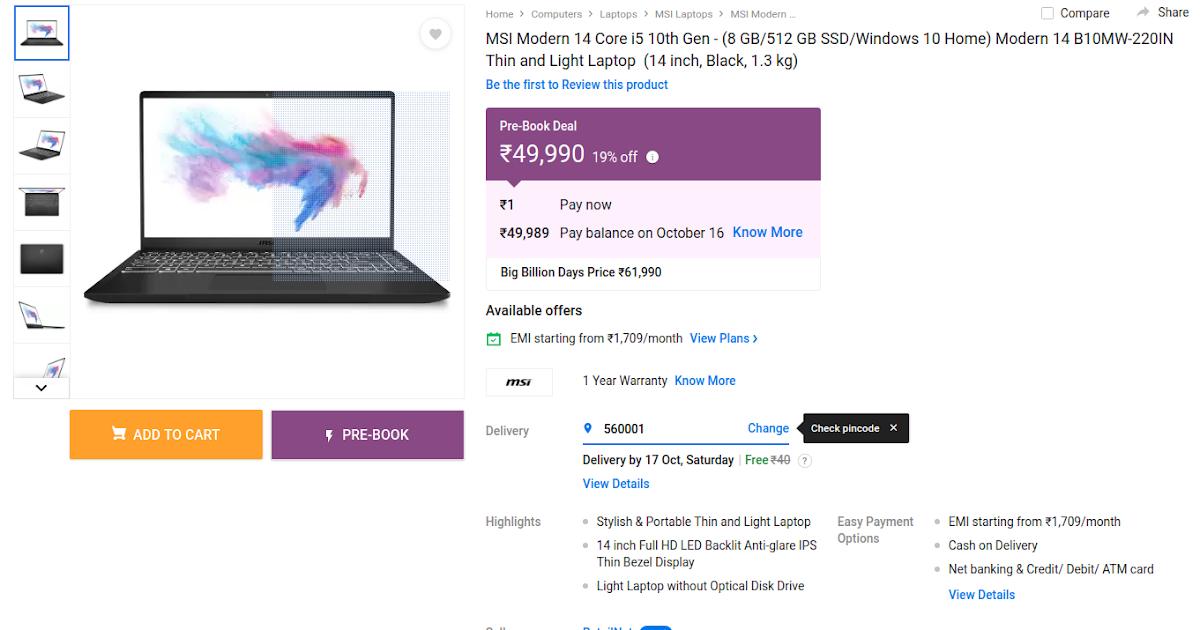**Detailed Caption:**

A detailed screenshot from an online store displaying the product page for an MSI Modern 14 laptop. The laptop is black, with a 14-inch display showcasing a vibrant blue and pink swirly artwork design on a white background. The product page features seven small thumbnail images on the left side, providing various angles and views of the laptop. 

Key navigation options such as "Home," "Computers," "Laptops," "MSI Laptops," and "Compare" are visible at the top. Below these, sharing options and the option to be the first to review the product are displayed. The product title reads "MSI Modern 14 Core i5 10th Gen 8GB 512GB SSD Windows 10 Home, Modern 14 B10 MW-220IN Thin and Light Laptop." 

The laptop is priced at $49,990, after a 19% discount from the original price of $61,990. A deal is available with an immediate payment of $49,989 and the balance due by October 16th. Prominent buttons show options to "Add to Cart" with an orange background and "Prebook" with a purple background.

Details indicate that the laptop is lightweight at 1.3kg and lacks an optical disk drive. Additional information highlights features like the sleek, portable design, and a 14-inch screen. Available payment methods include cash on delivery, net banking, debit cards, credit cards, and installment plans starting from $1,709 per month. Delivery details promise free shipping by October 17th, with options to change the delivery area code. An MSI one-year warranty is also mentioned.